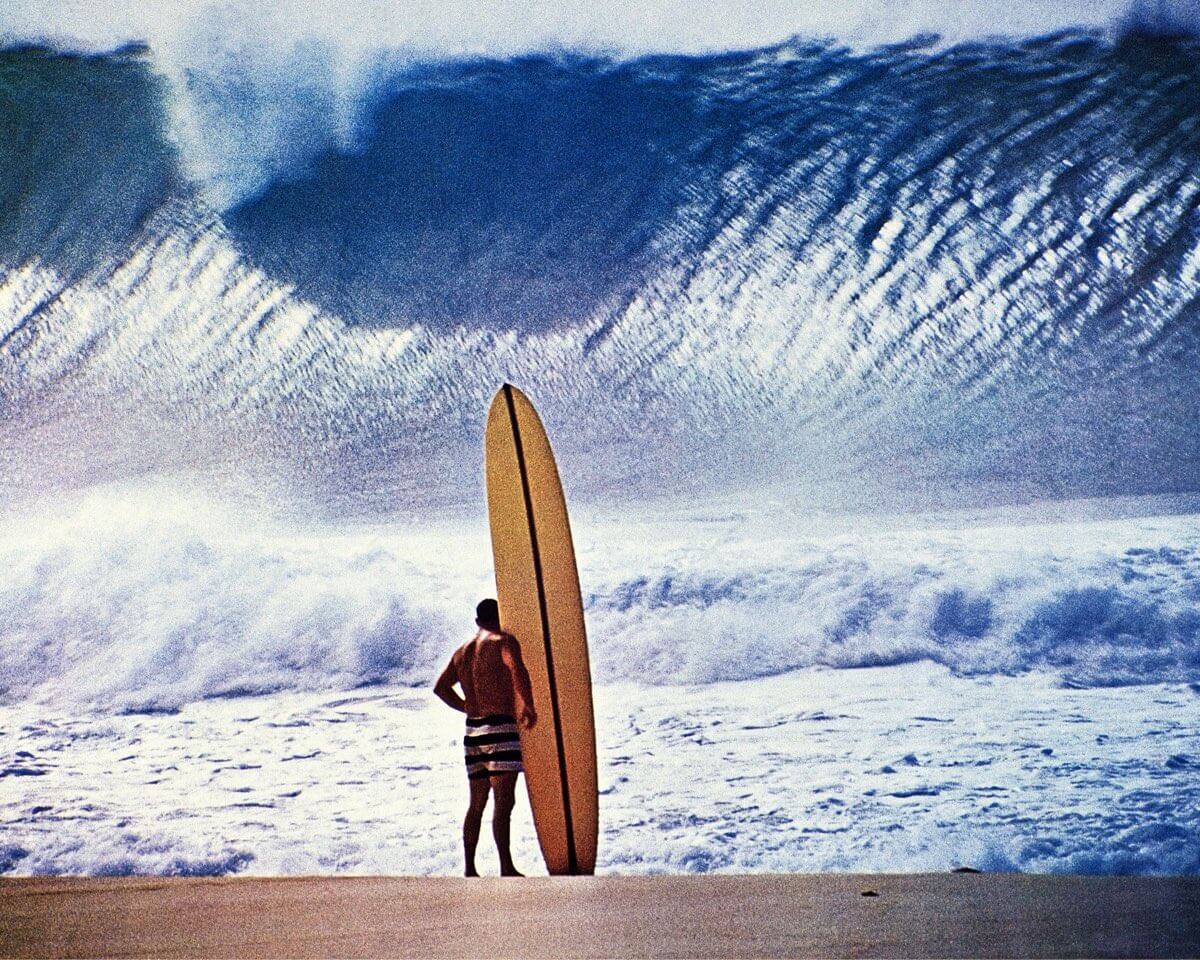This grainy, vintage-looking photograph captures a solitary, muscular Caucasian man standing on a sandy beach, facing the ocean. The man, who appears to be a surfer, has tan skin suggesting he spends a lot of time at the beach. He is wearing outdated tan and black horizontally striped swim trunks. Beside him stands a large, creamy-yellow surfboard with a central black stripe, propped up vertically in the sand. The man gazes out at the ocean, where massive, turbulent waves—towering at an estimated height of roughly 60 feet—loom ominously in the background, poised to crash dramatically. The beach itself is a brownish hue, and the entire scene is tinged with a sense of impending danger due to the disproportionately large waves, suggesting the sheer power of nature that the lone surfer is about to face. The overall grainy texture of the image adds an element of nostalgia and highlights its likely age.